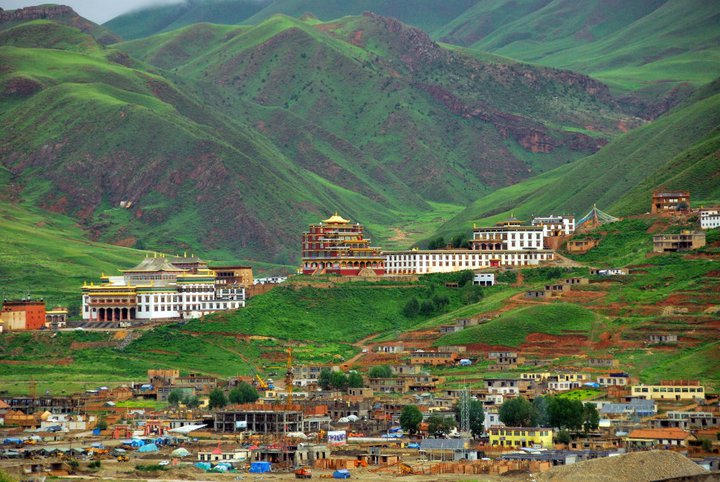The image captures an overhead view of a picturesque village nestled in a mountainous, lush green landscape. The village features an array of low-rise buildings, primarily topping out at three stories. The architecture includes smaller one-story homes with open windows and larger, potentially administrative or religious, structures distinguished by their white façades, sloped roofs, ornate gold accents, and red arched windows. Notably, a building left of center is under construction, its unfinished frame visible. The scene is set in daylight, bathing the vibrant green hills, trees, and terrain in natural light. The predominant colors are light green, brown from roofs, and the occasional red and white detailing, all contributing to the serene, natural beauty of this mountaintop settlement.